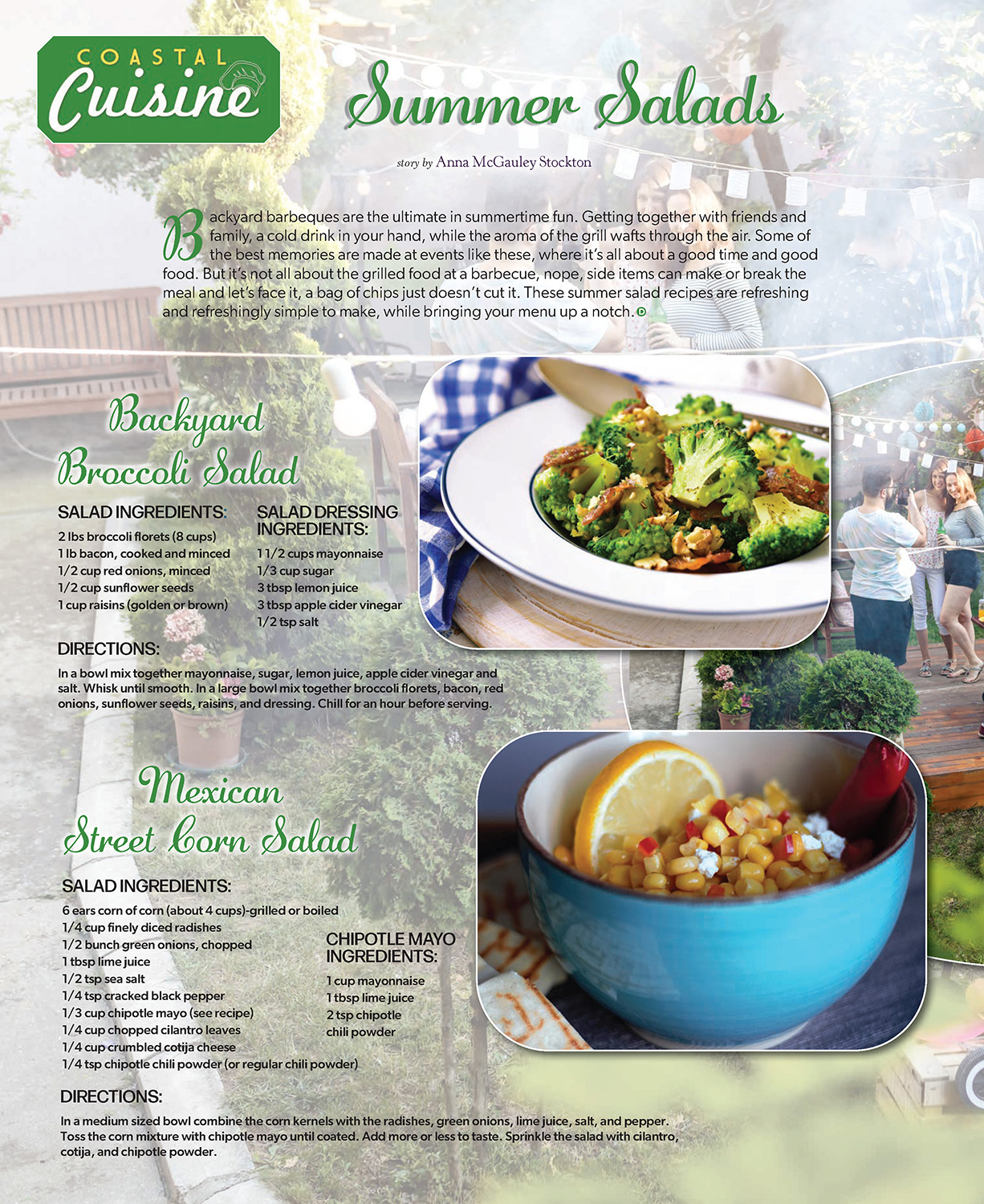This image from the website Coastal Cuisine features an infographic on summer salads, with the story by Anna McCauley-Stockton. The image is vertically rectangular, devoid of a border, and includes some digital enhancements. The background shows an outdoor setting with trees, a lawn, a sidewalk, flower pots with pink flowers, and people dancing and partying. The top left corner of the infographic has a green square with the Coastal Cuisine logo in white and green, featuring the word 'coastal' in yellow. 

A large green cursive text across the middle announces "Summer Salads," introducing two detailed recipes. The first, the Backyard Broccoli Salad, is depicted with an image of a white bowl with a blue trim, filled with broccoli and meat. Adjacent text includes a description of its ingredients and directions. The second recipe is for Mexican Street Corn Salad, shown in a big blue bowl with corn, a slice of lemon, and a chili pepper. Similar to the first recipe, detailed ingredients and directions accompany the image.

The article begins with a narrative about the joys of backyard barbecues, emphasizing that side items, like these summer salads, are essential for enhancing the dining experience. Throughout the infographic, multiple images and paragraphs provide a comprehensive guide to preparing these refreshing and simple summer salads.